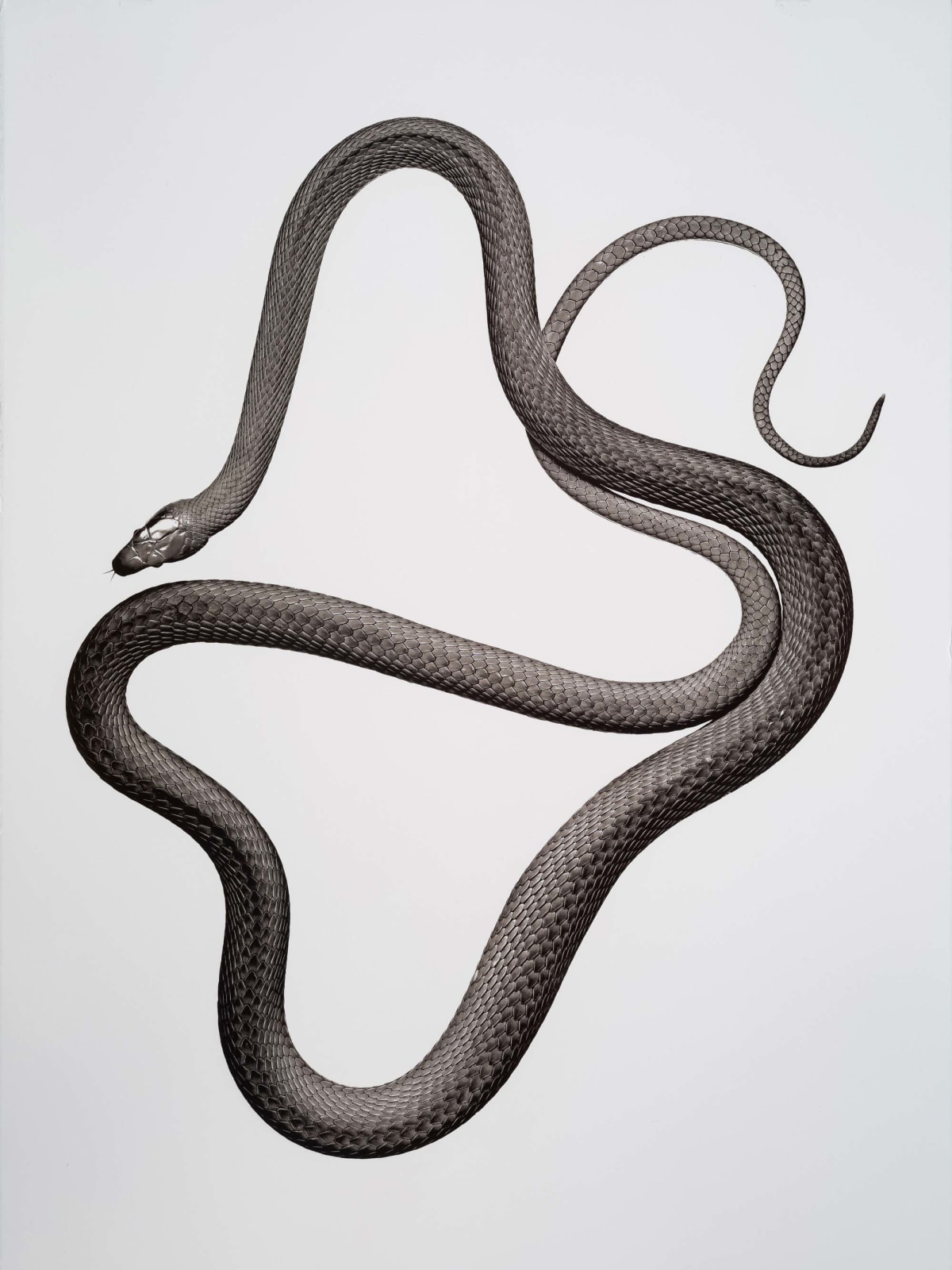This image showcases a detailed 3D digital render of a snake, characterized by its sleek, dark gray coloration against a light gray backdrop. The snake's body, slightly shiny and revealing its scale texture, is intricately coiled in an intricate pattern. Its head, featuring reflective, less scaly areas, is positioned on the center left, while its tongue protrudes and gray eyes are discernible. The snake's lengthy body creates a complex shape, curling up toward the top left and forming a sideways heart shape, looping down toward the center right. It then descends to the bottom center left, coils again almost touching its head, and returns to the center right, forming an 'S' shape before looping beneath and into another coil. The overall composition highlights the snake’s coiling length and detailed features against the contrasting backdrop.